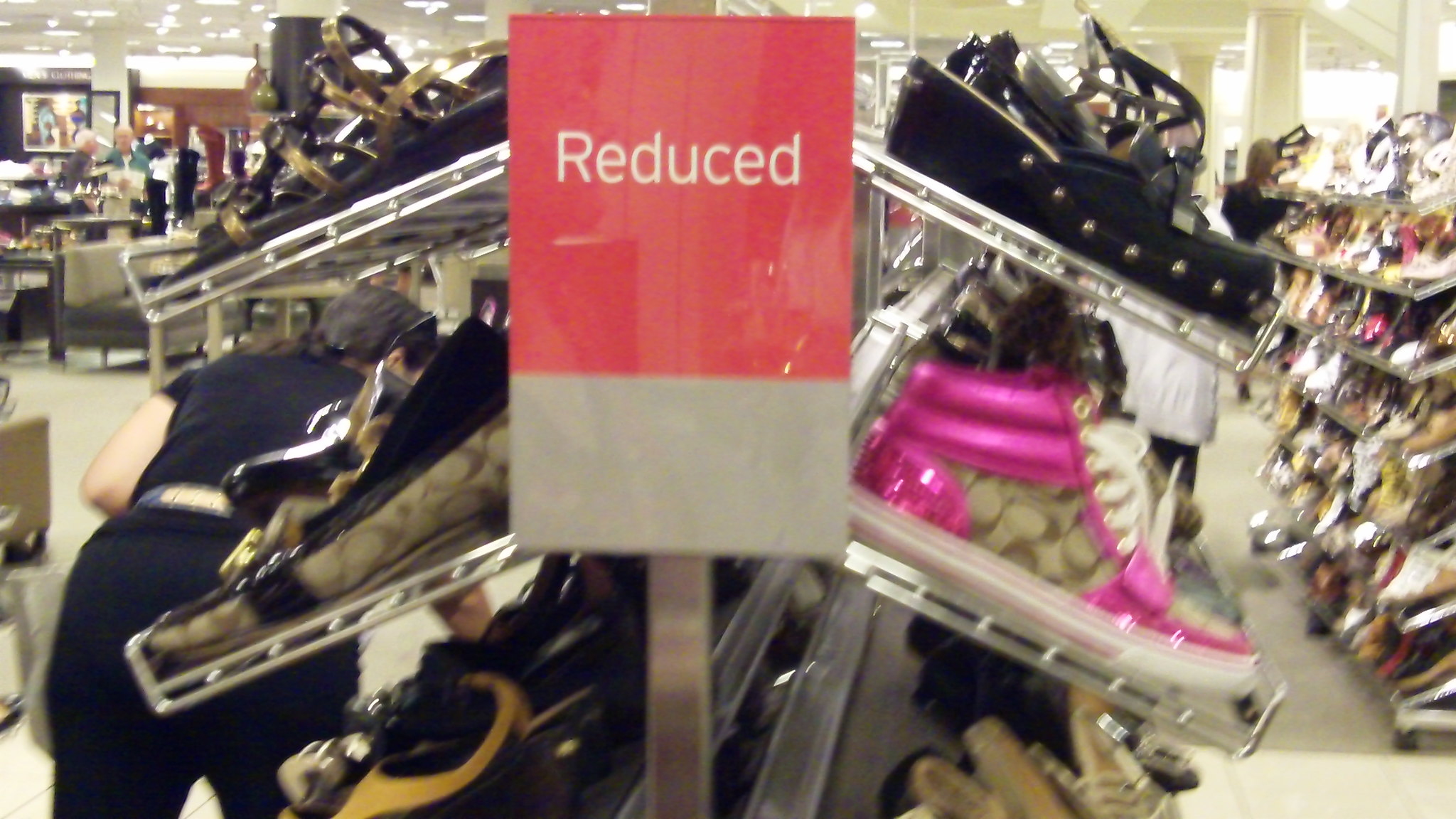This image captures the interior of a retail store, focusing on a silver metal shoe rack prominently positioned in the frame. The top of the rack features a distinct rectangular sign with a gray lower third and a red upper two-thirds, emblazoned with the word "reduced" in white, lowercase lettering except for the capital 'R'. The rack is laden with a variety of shoes displayed on both sides, angled slightly downward. Notable among them are a pair of high-top Coach sneakers with hot pink accents, a tan Coach print, sparkly heels, and white laces positioned on the right side, and another slip-on Coach shoe on the left side with a dark stripe. Gold Grecian-style flat sandals and black sandals with studs are also visible. Surrounding this central rack, various shoppers explore the selections; one individual with dark hair is bent over examining the shoes, while another dressed in white stands nearby. The blurry backdrop includes more shoe racks, ceiling lights spanning from left to right, and a hint of furniture or additional clothing items in the upper left corner, along with some scattered chairs and wall decorations.